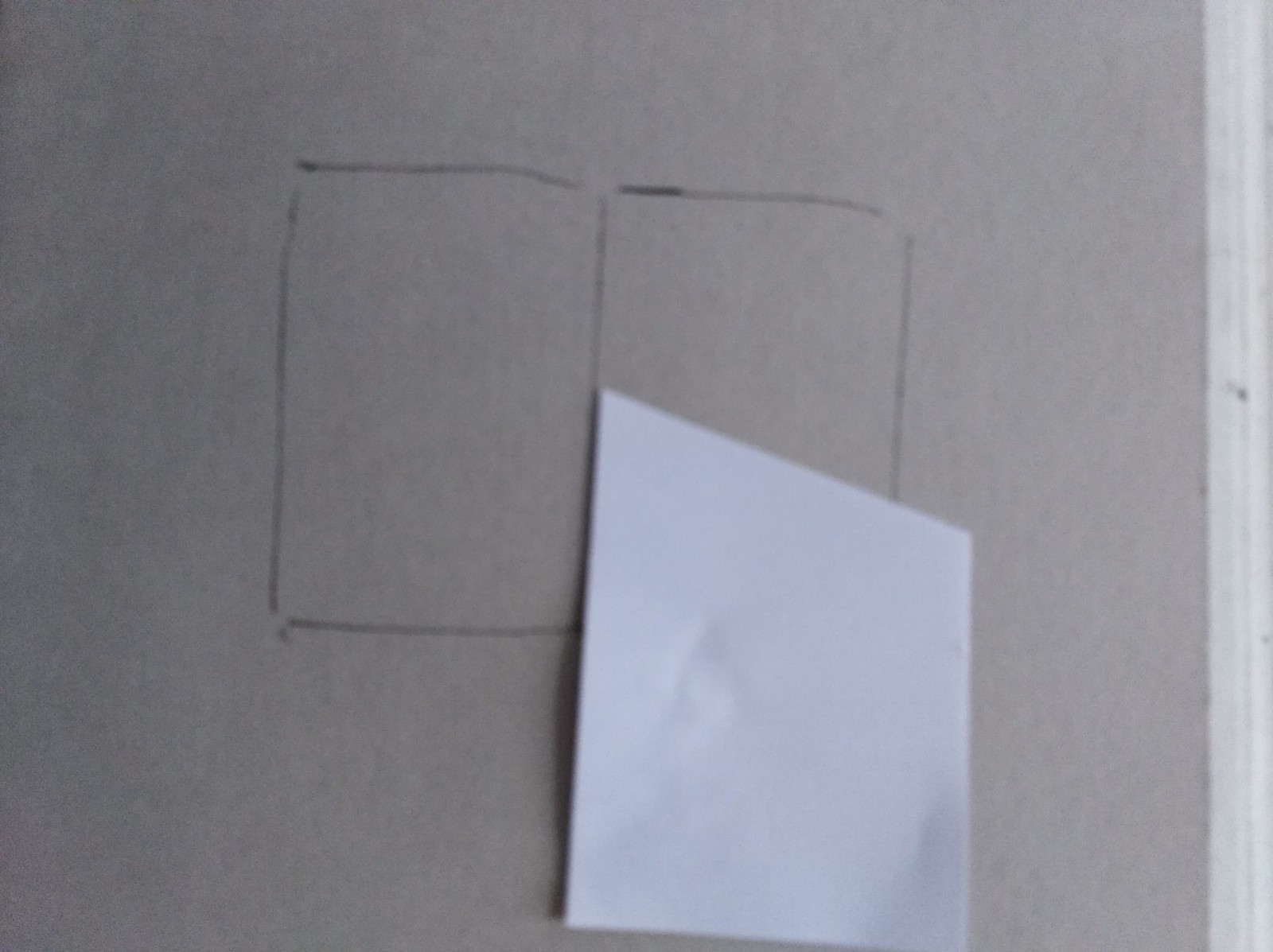In the image, a nondescript surface serves as the backdrop for a simple pencil drawing, likely on a table. The drawing comprises a rectangular box bisected by a single vertical line, reminiscent of an open book but much more rudimentary. On top of the drawing, a plain white piece of paper, folded into a rhombus shape, lies flat. The paper is unmarked, its creases clearly visible. The overall simplicity and lack of context create an enigmatic scene, leaving much to the viewer's interpretation.